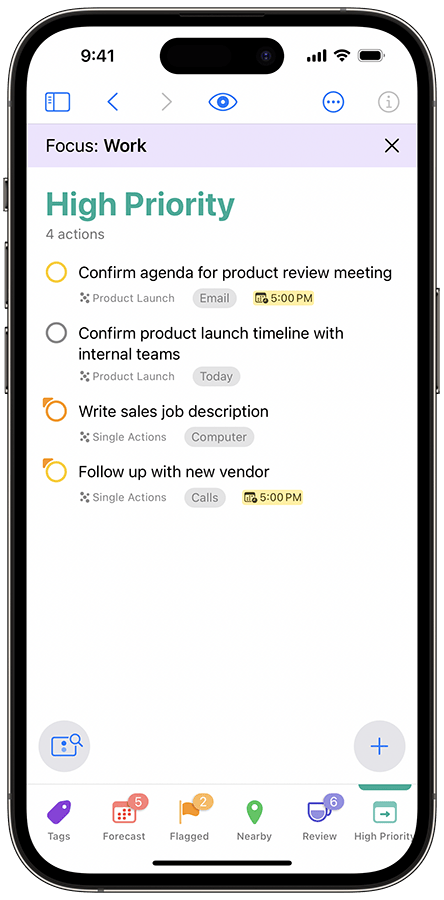The image depicts a mobile device, though the exact model is indistinguishable—it could be an iPhone, Samsung, or Google phone. The screen shows a detailed reminder list under the header "Focus Work," which is highlighted by a prominent purple bar at the top. This list specifically categorizes reminders marked as "High Priority," with the term "High Priority" distinctly written in green for emphasis. 

The first reminder on the list is to "Confirm agenda for product review meeting at 5:00 PM." Following this, the second reminder states, "Confirm product launch timeline with internal teams." The third task is to "Write sales job description," and the fourth reminder is to "Follow up with a new vendor," which is also scheduled for 5:00 PM.

Along the bottom of the screen, various general function buttons are visible, including tags such as "Tags," "Forecast," "Flag," "Nearby," "Review," and "High Priority," allowing for efficient navigation and organization within the application.